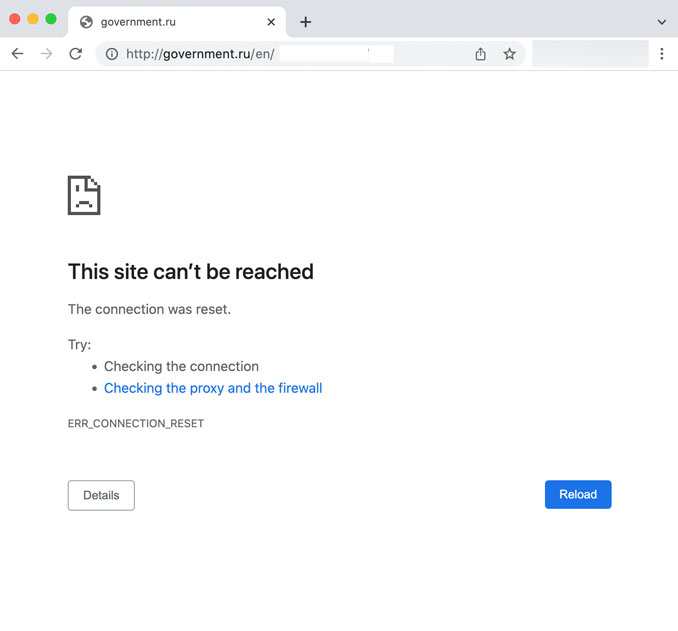The image is a screenshot taken from a computer browser showing an error on a webpage. At the top of the browser window, there is a white tab labeled "government.ru" followed by the address "http://government.ru-en." Below this, the main content on the screen displays a white background resembling a piece of digital paper, with the top right corner dog-eared. In the center of this digital paper is an illustration of a single, circular eye paired with a frowny face.

The main text in black reads, "This site can't be reached." Directly underneath, a subtext states, "The connection was reset." Further down, there are two bullet points suggesting actions to resolve the issue: "Checking the connection" and "Checking the proxy and the firewall." 

At the bottom of this section, an error code "ERR_CONNECTION_RESET" is displayed, followed by two buttons. The first button, framed with a gray outline and black text, is labeled "Details." The second button, filled with blue and featuring white text, is labeled "Reload."